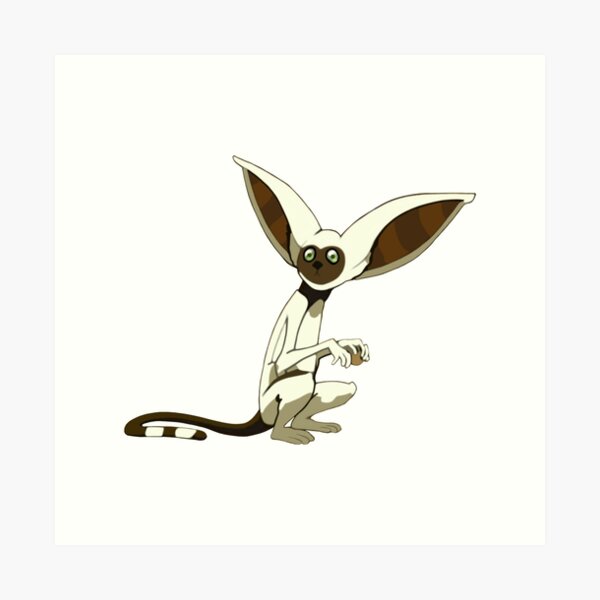The image depicts a whimsical, animated creature set against a predominantly white background. The composition features an off-white square framing a smaller, white square, creating a layered backdrop. The creature itself is a unique blend of various animal characteristics. It has large, bunny-like ears with inner sections that are striped in shades of brown and light brown. The majority of the creature’s body is white, contrasting with its dark brown tail, which is long like a rat’s and adorned with two distinct white spots. Its eyes are green, each with a black pupil, and it possesses the face of a mouse, though intriguingly lacking whiskers. The creature's legs are bent and elongated, resembling those of a kangaroo, as do its arms, further enhancing its fantastical and composite appearance.